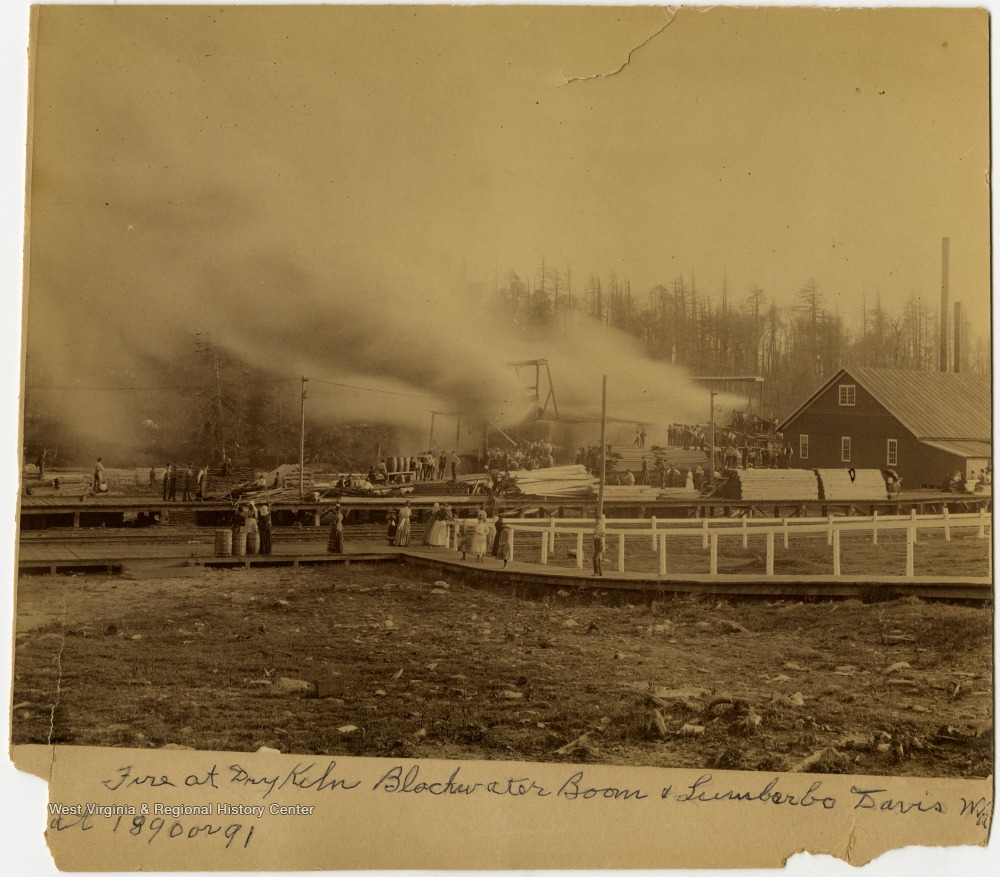This postcard-like, sepia-toned photograph from 1890 or 1891 captures a devastating fire at the "Dry Kiln, Blackwater, Boom, and Lumber Company" in Davis. The sky above, a dull peach hue, is choked with thick clouds of smoke billowing from multiple wooden structures engulfed in flames. In the foreground, a worn dirt field leads to a wooden walkway or boardwalk, which is strewn with debris and flanked by stacks of lumber and scattered barrels. 

Onlookers, including women in long dresses and children in gowns and caps, stand in somber clusters, etched against the burning backdrop. Men, some possibly attempting to douse the flames with water, can be seen nearer to the heart of the inferno. Behind the chaos, tall pine trees frame the horizon, partially obscured by the pervasive smoke.

The image is annotated at the bottom with black cursive writing that specifies the event and date, now faded and partially torn, and is additionally labeled in print: "West Virginia and Regional History Center." The historical gravity of the scene is intensified by the eerie absence of modern firefighting equipment, marking a poignant moment in time captured for posterity.